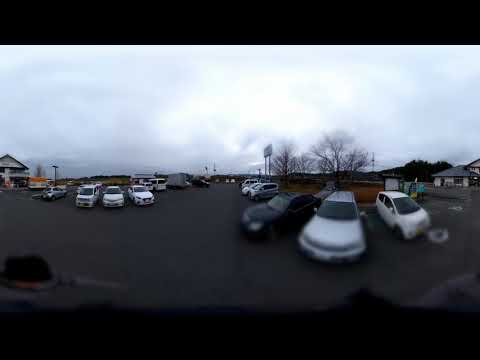The image is a panoramic, horizontally aligned, rectangular picture with a solid black border at the top and bottom. Captured from inside a car, the perspective reveals a parking lot on an overcast, possibly rainy day, with raindrops dotting the lens. The scene encompasses multiple cars, vans, and trucks parked in strips. Brown grass and leafless trees suggest it's winter, further accentuated by the stormy weather. Houses, both older two-story and single-story, line the background, flanking the parking lot, which includes a small island filled with mulch. A tall, white billboard, though illegible, marks the lot’s entrance, and a large white building stands opposite, surrounded by more parked vehicles. The sky is predominantly gray, with the occasional hint of bright white, underscoring the cloudy day.